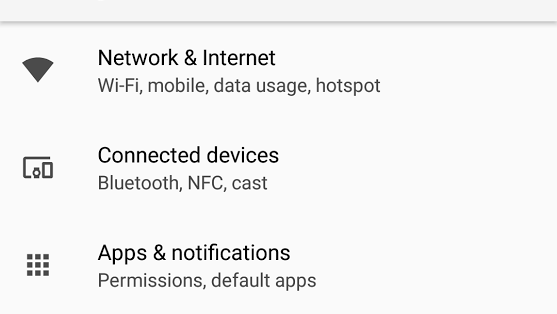The image showcases a section of a smartphone's settings menu against a light gray background. At the very top, a horizontal dark gray line stretches across the image. Below this line, three different settings categories are listed:

1. **Network & Internet**: This section includes options for Wi-Fi, mobile data usage, and hotspot. Accompanying this is a solid black Wi-Fi icon on the left side.
   
2. **Connected Devices**: This category encompasses Bluetooth, NFC, and CAST settings. To the left of this text is an icon that appears to depict a cell phone outline with a few signal lines, representing connectivity options.
   
3. **Apps & Notifications**: Under this category, you can find settings for permissions and default apps. The associated icon is a grid of nine small squares arranged in three rows of three, signifying the various apps.

Each of these sections includes detailed options pertaining to their respective functionalities.